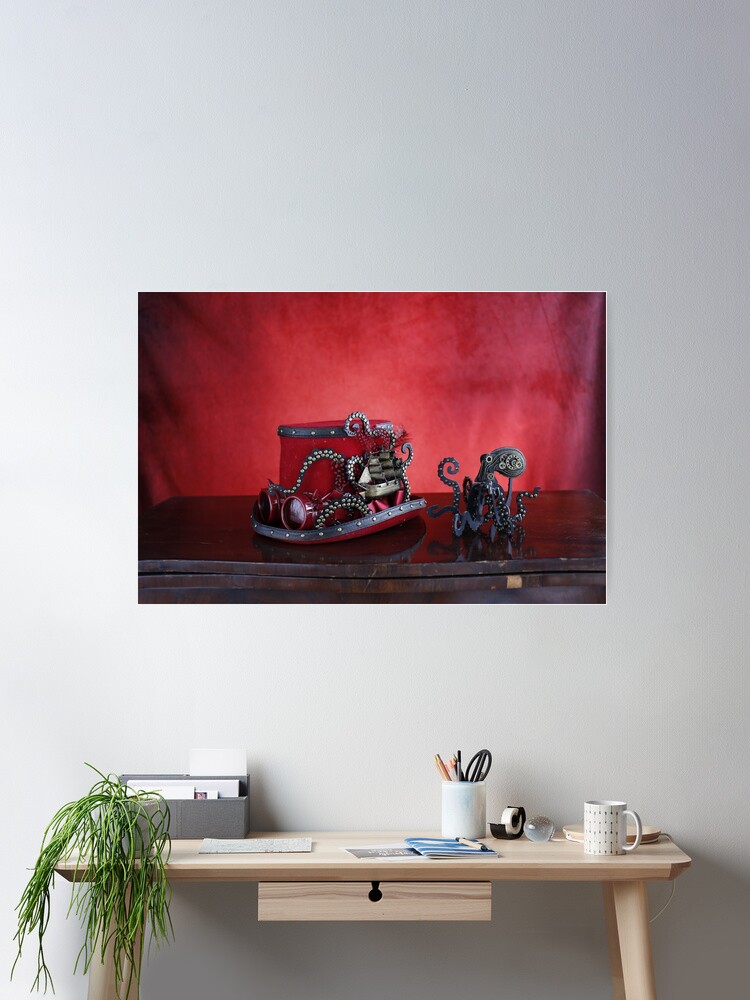The image depicts a pristine white wall in a minimalistic living room. Centered on the wall is an eye-catching piece of art with a rich red and burgundy background. The artwork depicts a steampunk-themed tableau featuring a red top hat adorned with dark gray goggles and a metallic octopus wrapping around it, alongside a dark gray statue of a squid on a brown table.

Beneath the artwork, there's a light beechwood desk with four legs and a flat surface. The desk has a small drawer underneath and is adorned with a variety of items: a white coffee cup, a mug filled with scissors and pencils, a tape dispenser, papers, and a white lamp with an extended arm. A small potted plant with trailing green ivy leaves is positioned to the side, adding a touch of nature to the tidy workspace.